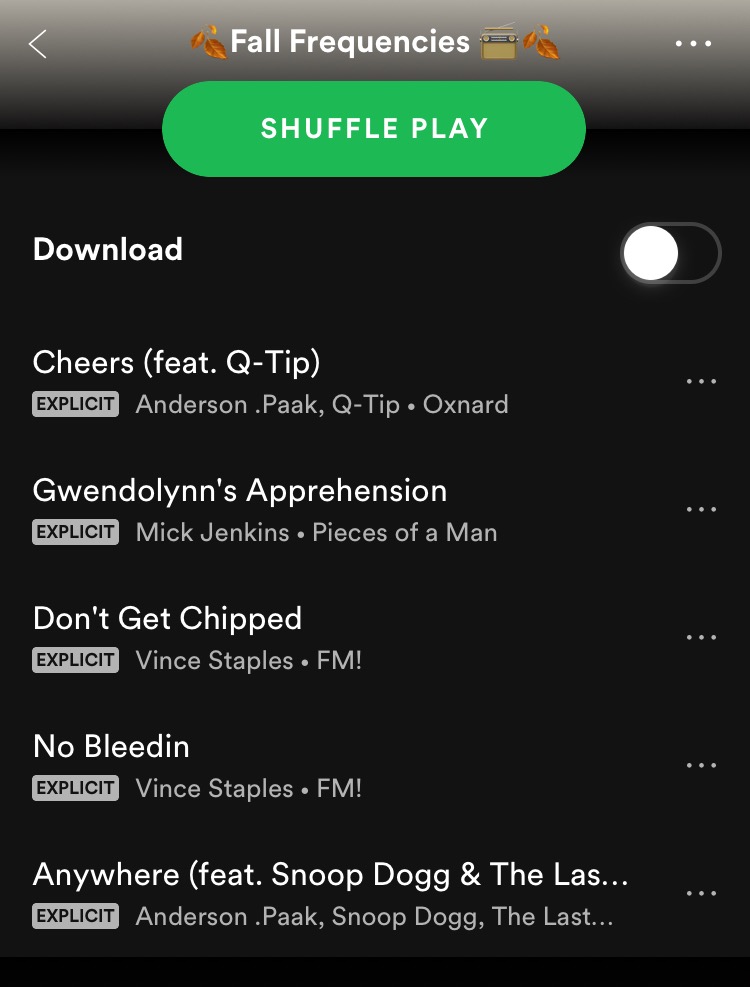Screenshot of a Mobile Application Interface:

The screenshot portrays a mobile application featuring a predominantly black background, with a gradient starting in the middle and transitioning from black to light gray towards the top header. Centered at the top of the header is the title "Fall Frequencies" in white text, flanked by an orange leaves emoji on the left, an old-fashioned olive-colored radio emoji in the middle, and another orange leaves emoji on the right. In the top corners, there are interface symbols: a white left-pointing arrow in the top left and three horizontally aligned white dots in the top right.

Below the title is a prominent, green pill-shaped button labeled "SHUFFLE PLAY" in large, all-caps white text. To the left of this button, the word "Download" appears in white text. On the right of the button, there is a selection toggle that consists of a black pill shape with a white circle on the left side and a medium-width light medium-gray outline around it.

Further down, the interface displays lists of songs and information. Each list entry includes the following elements: a white, left-justified title; beneath the title, an all-caps "EXPLICIT" label inside a light gray box with rounded corners; to the right of this label, in light gray text, is the name of the artists, separated by light gray dots; and to the far right, three horizontally aligned light gray dots, justified right.

An example entry reads:

- **Cheers (feat. Q-tip)**
  - Anderson, DotPak, Q-tip, Oxnard
  
The layout and design elements deliver a cohesive and user-friendly interface for music navigation.